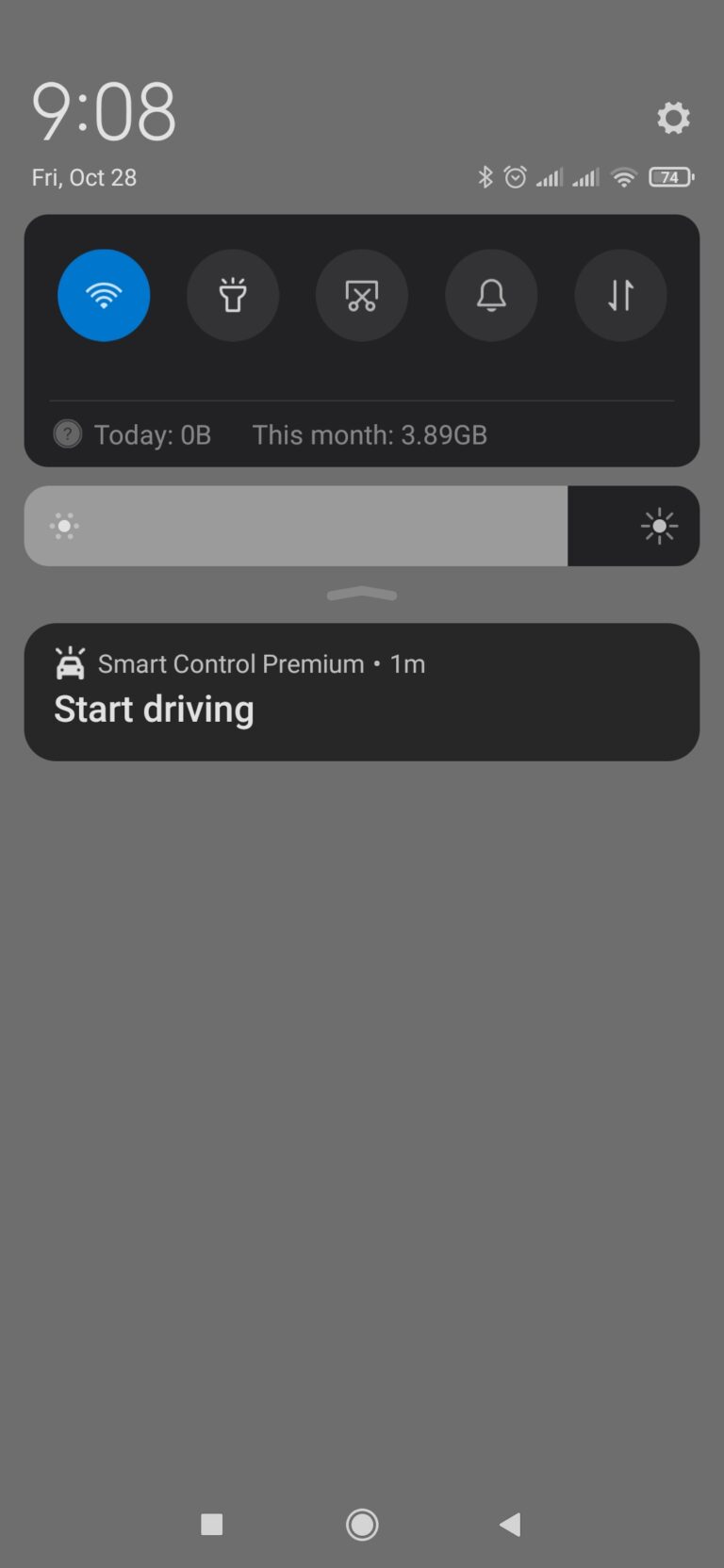The image depicts a screenshot taken from a mobile device. The predominant background color is gray with white text, and there are also elements in black and blue. The screenshot was captured at 9:08, as indicated by the large white font displaying the time. In the top right corner, a white gear icon for settings is visible. Other icons on the status bar include the Bluetooth icon, an alarm icon, and the carrier signal for mobile data, all in white. The device is connected to Wi-Fi, and its battery life is at 74%.

Further elements displayed near the top of the screen include a blue circle icon representing Wi-Fi, a flashlight icon, a mail icon, and an alarm bell icon, all set against a blue background. The text "Today 0B" signifies no data usage for the day, while "This Month 3.89GB" indicates data usage for the month. There is also a gray bar showing the brightness level of the phone's display.

The app "Smart Control Premium" is open, prominently displaying options related to driving. It includes a "Start Driving" button, along with record, stop, and back buttons. The overall layout and specific details lend the screenshot a structured and technical appearance.